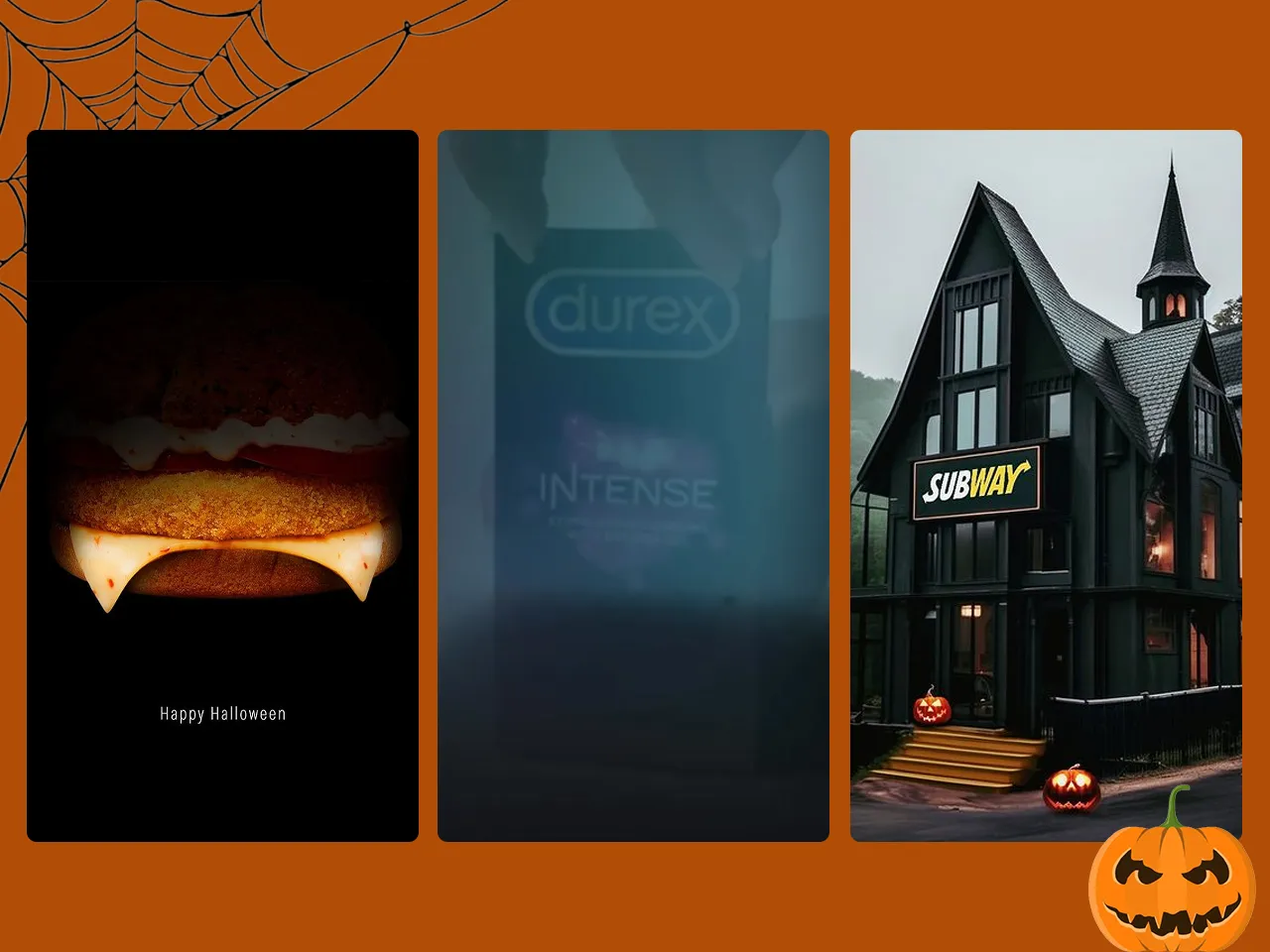The image features a dark orange background with a black spiderweb positioned in the upper left corner, setting an eerie Halloween atmosphere. Divided into three distinct long rectangles, the first section showcases a shadowy black background with a tantalizing centerpiece: a piece of chicken topped with melted cheese sprinkled with red specks, nestled on a bun. Below this, in striking white text, the phrase "Happy Halloween" adds a festive touch.

The second rectangle shifts to a mysterious blue hue, enveloped in a smoky, foggy ambiance. Dominating this section is the brand name 'Durex,' emblazoned inside a circle, with the word 'Intense' displayed beneath it, alluding to a heightened sensory experience.

The final rectangle depicts a large, ominous black house with a steeple-like roof, exuding a haunted house vibe. Four steps lead up to a porch adorned with illuminated jack-o'-lanterns, their yellow eyes and mouths glowing menacingly. Above the door, in a rectangular sign, the branding 'Subway' is divided into 'Sub' in white letters and 'Way' in yellow letters, adhering to the familiar Subway logo style.

At the very bottom of the image, a graphic of an orange pumpkin with a green stem is displayed. The pumpkin's eyes and mouth are rendered in black, complementing the Halloween theme intricately woven throughout the composition.